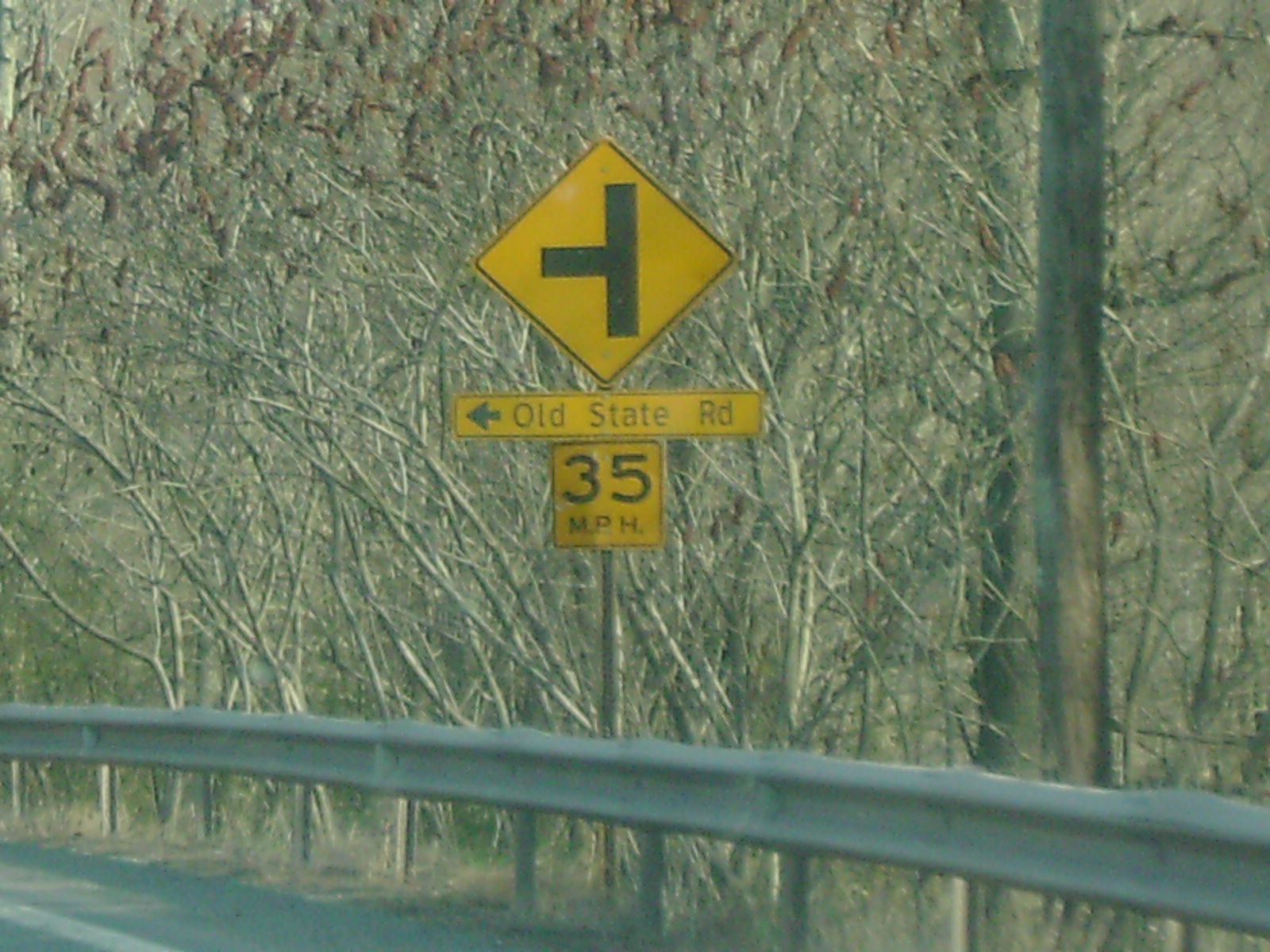This photograph captures a three-way intersection at a highway junction, with a secondary road approaching from the left. The viewpoint is from the curb, where a guardrail is prominently visible. A sign indicating a suggested speed limit of 35 miles per hour is present, specifically meant for the upcoming curve. An arrow points towards Old State Road, potentially placing this scene in Pennsylvania, although the tree backdrop evokes a distinctly New England landscape.

The season appears to be early spring or late fall, as evidenced by the bare branches of the trees and shrubs, including what seems to be sumac. Further into the background, more leafless trees stand against a clear sky, underscoring the transitional period of the year. In the lower left corner of the image, a road with a clearly marked stripe is visible, alongside another section of the guardrail. Additionally, the scene includes a utility pole and various scrubby trees or bushes, adding to the raw, unembellished charm of the location.